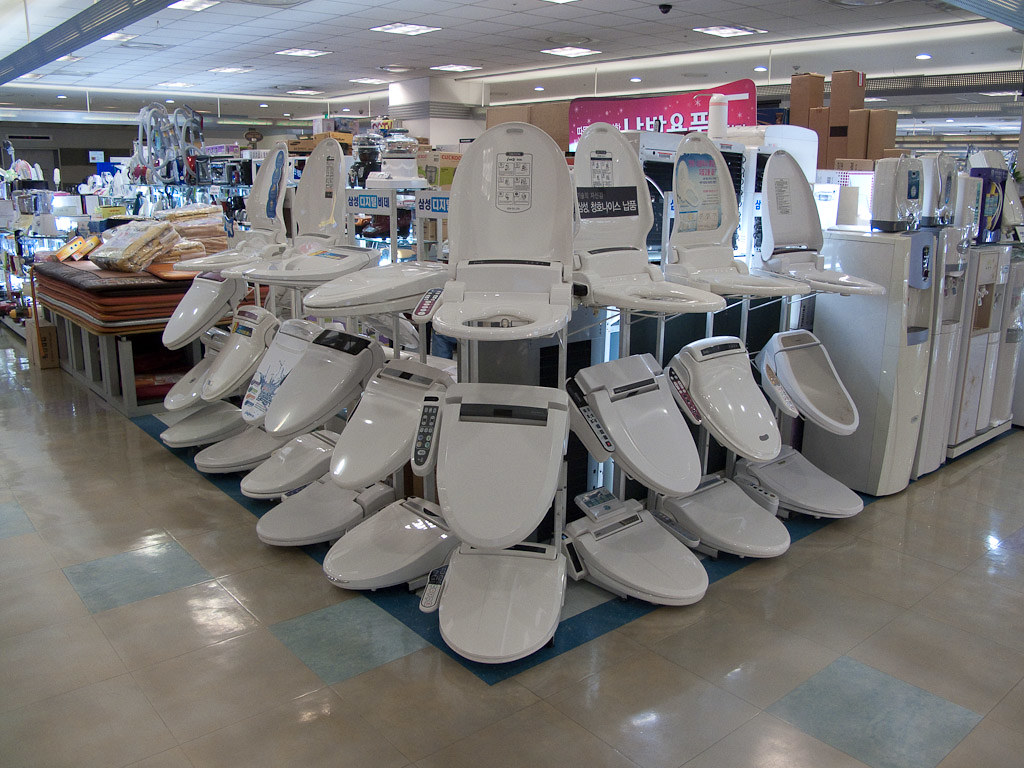This image captures the interior of a pristine, brightly lit Korean department store, showcasing a prominent display of various high-tech toilet seats. The seats, all gleaming white and some featuring buttons on their sides, hint at advanced functionalities. Surrounding this main display, the store's immaculate and well-organized layout is illuminated by bright fluorescent lights, enhancing the crisp, squeaky-clean ambiance. In the background, on the right, are compact water dispensers designed for large jugs, and on the left, neatly stacked towels, beddings, and possibly some rugs can be seen. The signage throughout the store, adorned with Korean text, confirms the store's location. A closer look reveals additional boxed items meticulously arranged, contributing to the warehouse-like atmosphere of this comprehensive appliance and home goods retailer.